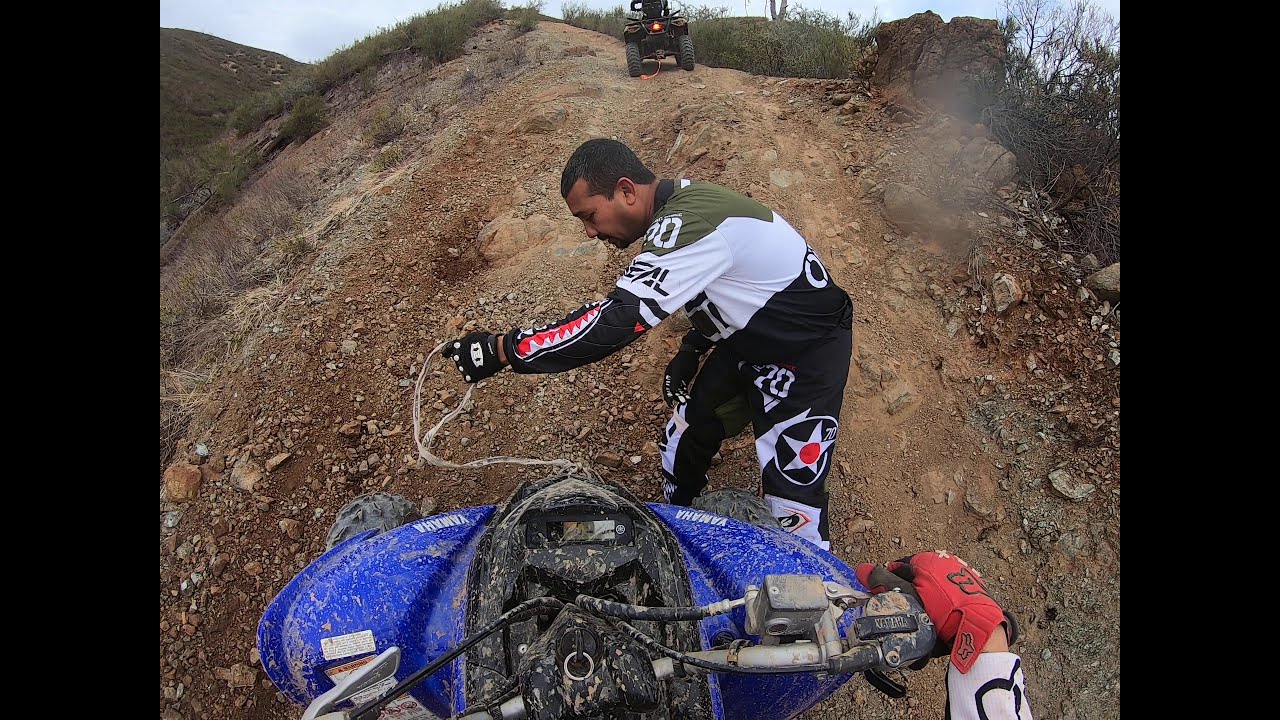The image, framed by tall black vertical borders on each side, captures a dynamic scene from the point of view of a rider on a blue ATV, which is heavily caked in mud. The rider's right hand is gripping the black and silver handlebar, adorned with a red glove and a white sleeve. Ahead, on a rocky, uphill dirt road, a man with dark hair is holding a frayed rope. He is dressed in an outfit comprised of black pants with a star on the leg and a green, white, and black shirt. This man appears to be attempting to pull or guide the ATV uphill. In the distant background, another ATV, perceived as a black three-wheeler, is parked at the top of the hill with a rope trailing behind it, hinting at a previously broken connection. Sparse grass, shrubs, and a bit of dust flying up add to the rugged and barren landscape of the uphill dirt road.